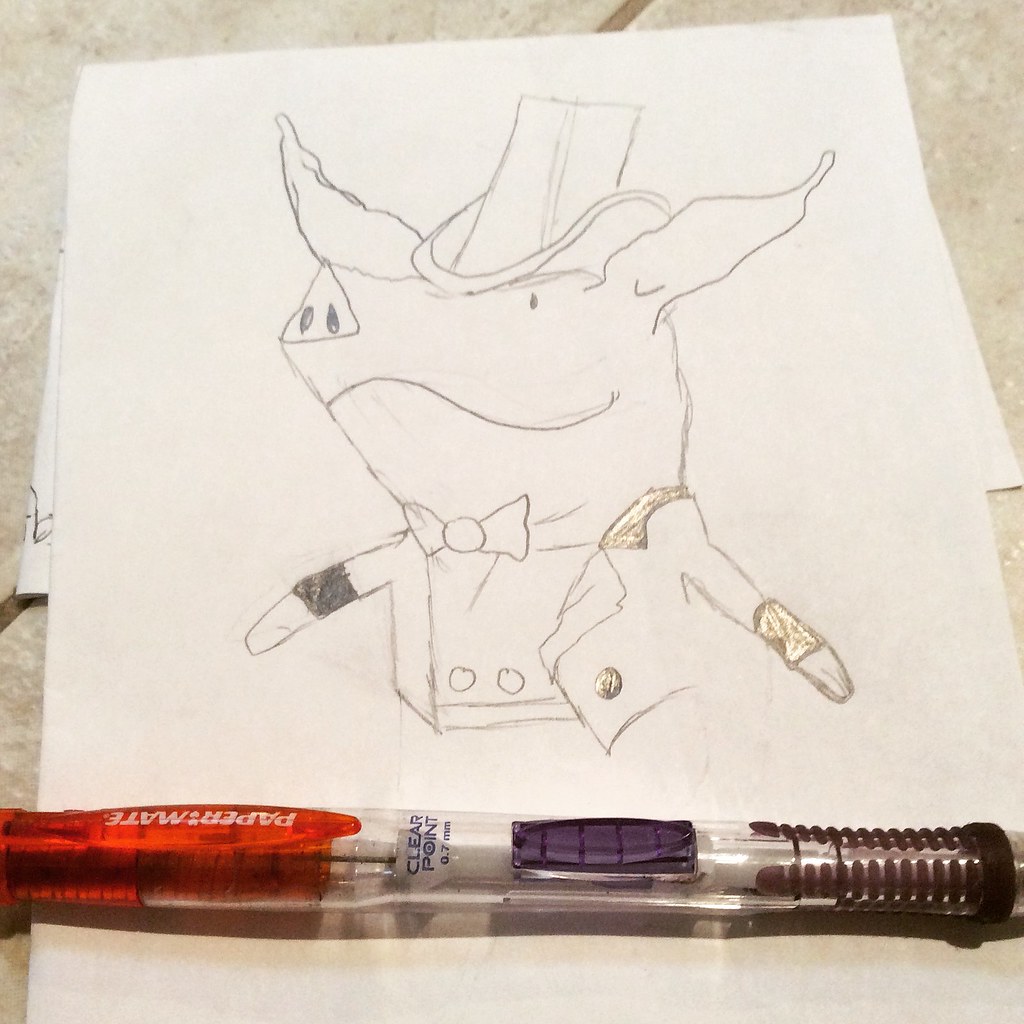The image features a white page from a sketch pad placed against a background of gray floor tiles. The drawing on the paper depicts a pig, which appears familiar, possibly resembling a character from a cartoon like those by Worthy Kids. The pig is looking to the left and is dressed in a distinguished and quirky ensemble. He sports a top hat and a bow tie, complemented by what looks like a blue jean jacket adorned with shoulder pads and a silver button at the bottom. An ink pen lies at the bottom of the paper; it features a red upper section, a clear middle, a blue button at the top, and a black grip at the bottom.